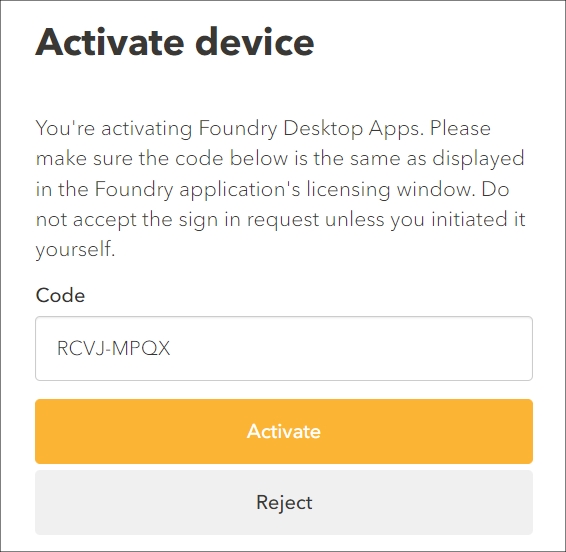The image features a user interface for activating a desktop application, set against a white background framed by a thin black border. At the top, in large, bold black text, there is a heading that reads "Activate Device." Below this, smaller black text provides instructions, stating: "You're activating Foundry Desktop Apps. Please make sure the code below is the same as displayed in the Foundry Applications Licensing window. Do not accept the sign-in request unless you initiated it yourself."

Further down, "Code" is prominently displayed in bold, black text. Beneath this label, enclosed in a large, rectangular, rounded-edge white box with a gray border, is a code in uppercase black text: "RCVJ-MPQX."

Below the code, there are two action buttons. The first is a rectangular button with rounded edges, featuring a vibrant orange background and white text that says "Activate." The second button, similar in shape but with a gray background, has the word "Reject" in black text.

Overall, the image appears to be a pop-up page guiding users through the activation process of a desktop application.